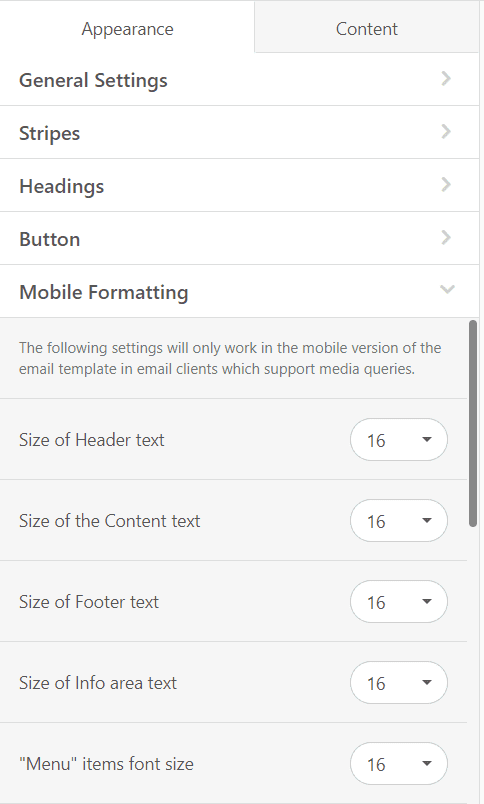The image depicts a user interface (UI) for customizing the appearance and formatting of an email template, with a specific focus on mobile settings. At the top right corner, the word "Appearance" is prominently displayed. Nearby, "Content" is also visible. Below these sections is a navigation bar labeled "General Settings". 

In the main settings area, there are options related to "Stripes", "Headings", and "Button". Additionally, a "Mobile Formatting" section and a dropdown menu are evident. A note clarifies that the following settings will only apply to the mobile version of the email template, as email clients that support media queries will implement these changes.

Further options allow users to adjust the size of various text elements:
- "Size of Header Text" with an input option showing a value of 16.
- "Size of Content Text" also set to 16.
- "Size of Footer Text" again appears with the value 16.
- A dropdown for "Size of Info Area Text", which is also set to 16.

A scroll bar is provided to navigate through these settings. At the very top of the pane, there are lines serving as dividers between sections, giving a clear organization to the different customizable areas. The UI seems designed to ensure seamless mobile rendering of the email, with specific features tailored for smartphone settings.